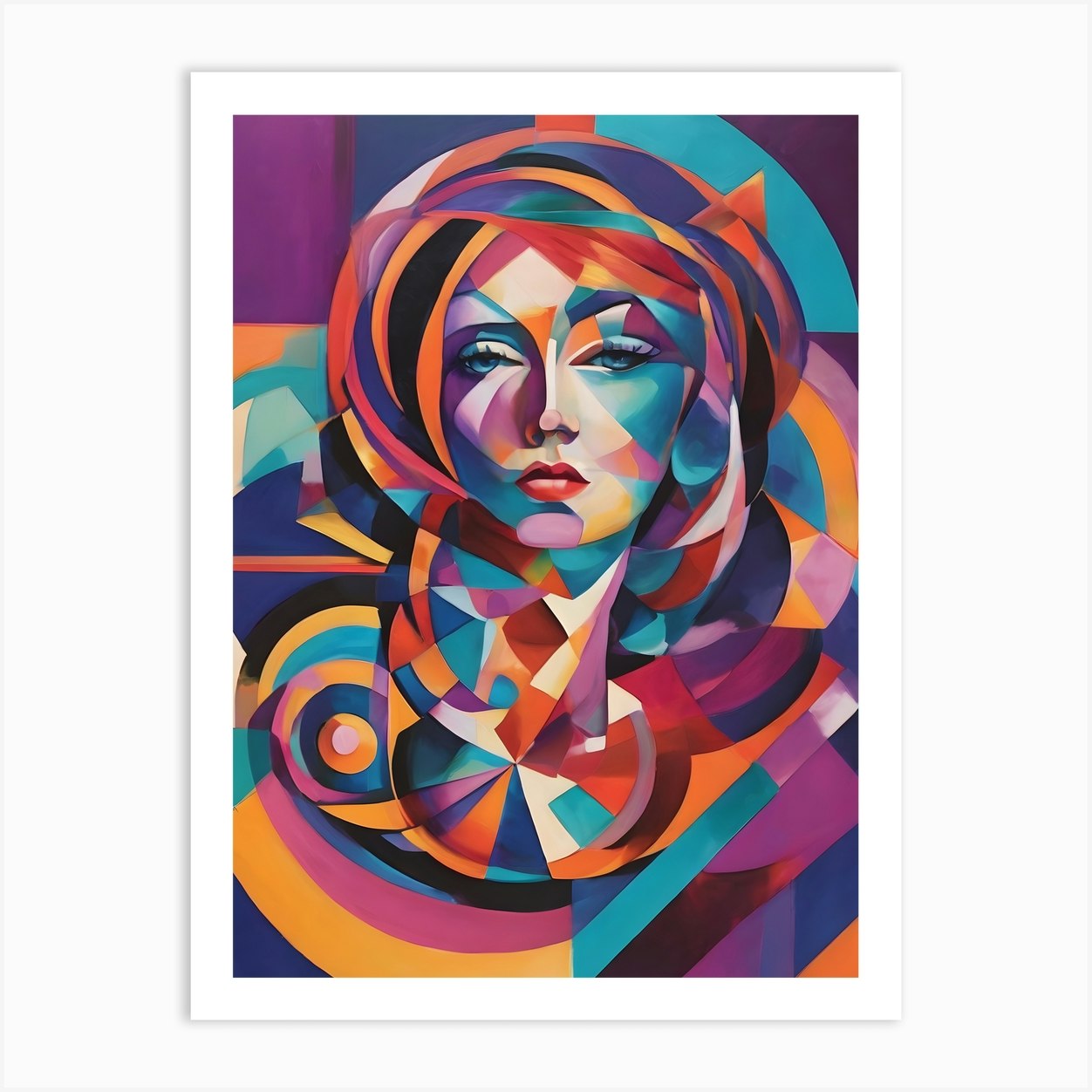The image is a vibrant, abstract portrait of a woman rendered in a striking array of shapes and colors. Framed by a sleek white border, this art piece—likely digitally or AI generated—features the woman's face as the focal point. Her sultry eyes, accentuated by long black eyelashes and blue irises, draw immediate attention. The woman has a delicate, thin nose bridge, small nose, and full red lips, with her chin depicted by a light purple circle. Her hair, which gives the impression of a turban due to the artistic style, adds to the exotic feel of the portrait.

The background and parts of her body are comprised of an eclectic mix of geometric shapes and a riot of colors, from purple, blue, and cyan, to variations of red, orange, and yellow, with touches of pink and magenta. Smaller shapes detail her facial features and body, while larger shapes create a dynamic backdrop, evoking a sense of movement and depth. The shapes around her range from squares and triangles to softer half-circles, further enhancing the abstract, modern feel of the artwork. The entire composition is imbued with a sense of organized chaos, with each color and shape harmoniously contributing to the overall captivating visual appeal.